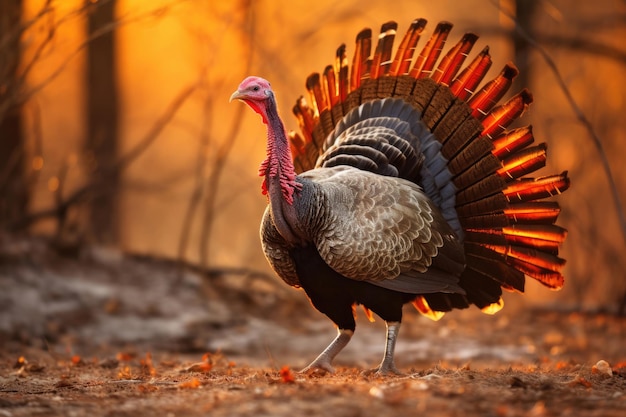The photograph captures a turkey standing outdoors on a dirt ground scattered with reddish leaves, in an area surrounded by thin trees particularly visible on the left side. The scene is suffused with an orange glow, likely from a setting sun, giving the image a warm, almost hyper-realistic effect. The turkey, facing left and occupying most of the right-hand side of the picture, has a distinctive appearance with a small head featuring pink skin, a yellow curved beak, and a neck that transitions from pink to gray with a reddish fringe. The turkey's long neck leads to a grayish chest, darkening under the belly due to shadows. The feathers on its wings are light brown with white tips, transitioning to gray and then brown, while its flared tail feathers shift from gray at the center to brown and reddish-orange. This creates a striking contrast against the illuminated background, highlighting the bird's intricate feather pattern. Additionally, despite the turkey's somewhat bored expression, the vivid and detailed plumage, combined with the soft focus and orange lighting, brings a unique liveliness to the photograph.